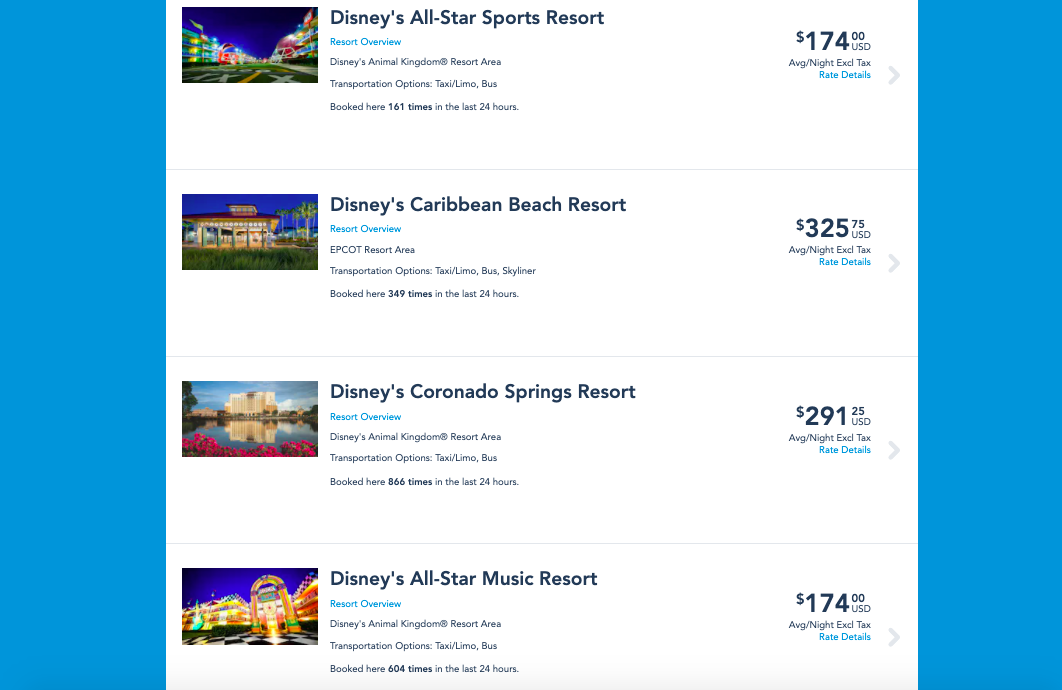### Descriptive Caption for Disney Resorts Screenshot

The image is a detailed screenshot of various Disney Resorts, featuring a blue background with a prominent white centerpiece. It highlights four distinct Disney Resorts along with their nightly rates and additional details. The resorts listed are:

1. **Disney All-Star Sports Resort** - $174 per night.
2. **Disney Caribbean Beach Resort** - $325 per night.
3. **Disney Coronado Springs Resort** - $291.25 per night.
4. **Disney All-Star Music Resort** - $174 per night.

The centerpiece of the screenshot is titled "Resort Overview" and provides information on the Disney Animal Kingdom and various transportation options available to guests. Additionally, it indicates the number of bookings for these resorts in the past 24 hours and includes images for each resort.

Each resort listing includes a small blue button labeled "Rate Details" which users can click to access more information about the respective resort. The overall layout is user-friendly, designed to give a comprehensive overview of the accommodation options and their pricing.